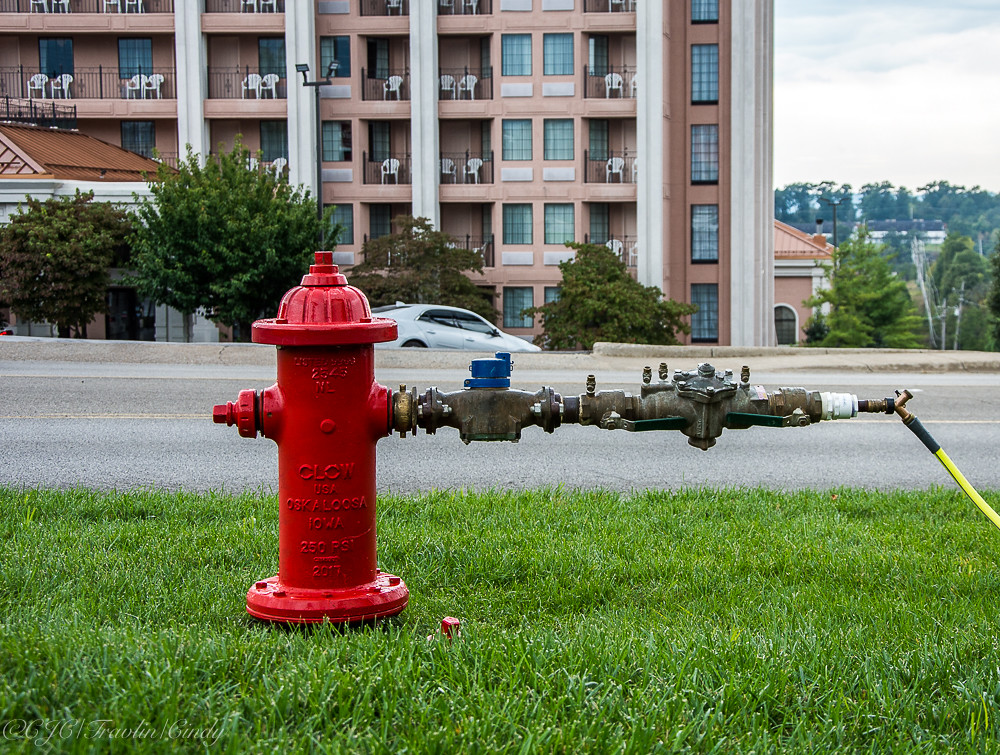In this vibrant daytime photograph, the focal point is a bright red fire hydrant situated in a lush green grassy lot. The hydrant features several brass fittings: one with a knob and two others with dual levers, eventually tapering to a small yellow garden hose attached to the smallest fitting. In the background, a paved road with a yellow stripe runs parallel to the scene, leading down a hill where a silver car is driving away. The right side of the image reveals more of the cityscape below.

Beyond the road, a prominent four or five-story apartment building with identical balconies catches the eye. Each balcony is adorned with two white resin chairs and two windows, suggesting uniformity, possibly indicative of a hotel. The building is set against a backdrop of various green trees, including palm and pine trees, bringing a touch of nature into the urban setting. The overall scene blends elements of urban infrastructure and residential hints, creating a detailed and dynamic street snapshot.